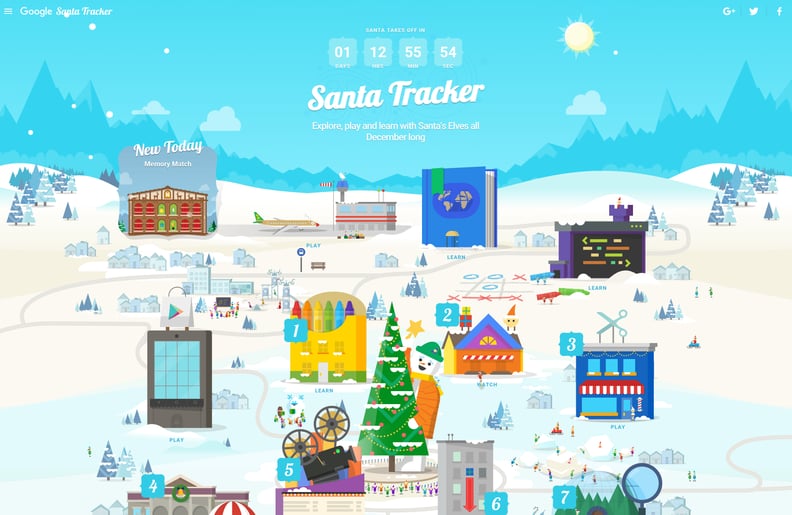The image showcases the Santa Tracker, an interactive feature available to explore, play games, and learn with Santa's elves throughout December. A prominent countdown reads "Santa takes off in 1 day, 12 hours, 55 minutes, and 54 seconds," displayed against a bright background featuring a large sun.

The scene includes a vibrant fountain and highlights new activities, such as a memory-matching game reminiscent of an advent calendar. An airport scene depicts an airplane preparing for takeoff, and there is an illustration of Earth in a giant book.

A tic-tac-toe game is being played in the snow with blue circles and red Xs, with a winning X marked by a line through it. Central to the imagery is a building designed to look like a box of crayons, with visible crayons in red, orange, yellow, green, blue, and purple.

A display resembling a smartphone screen is highlighted, and scene number four introduces a vintage-looking camera or projector, casting an image. There is a decorated Christmas tree adorned with pink ornaments and a snowman wearing a green hat and an orange coat nearby. On the far right, a building topped with a large pair of scissors signifies a barber shop.